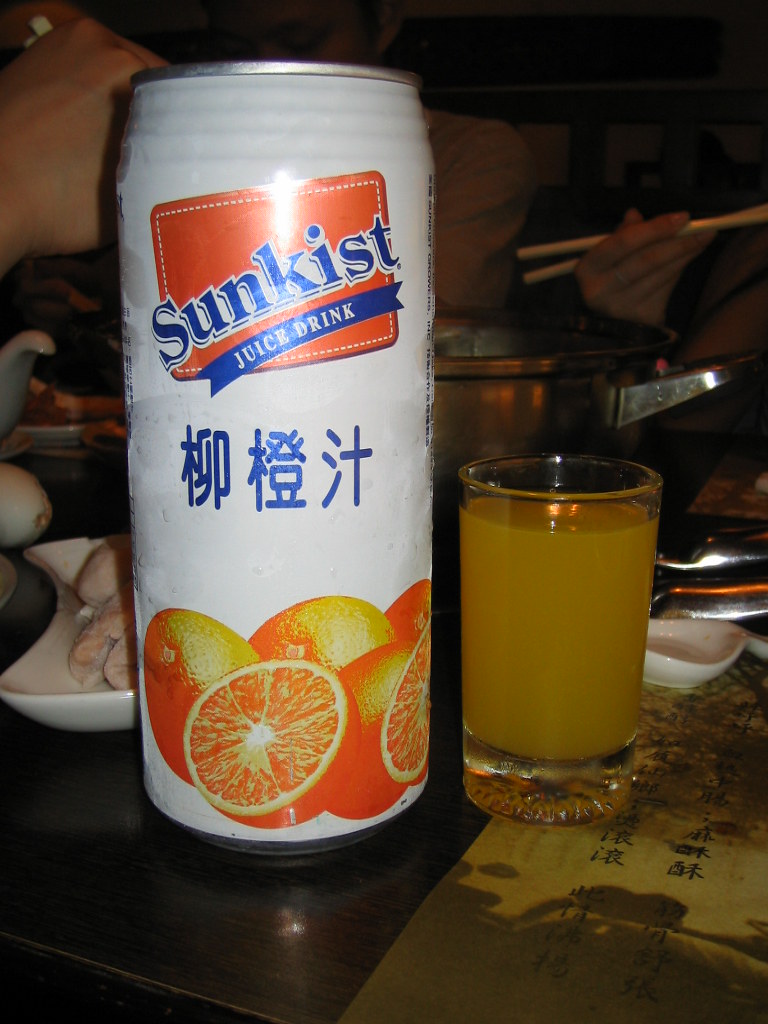A detailed photograph captures a refreshing scene: an aluminum can predominantly white in color, adorned with images of sliced oranges at its base. The can features a rectangular orange label with blue lettering boldly displaying the brand name "Sunkist" and the descriptor "Juice Drink" in white font on a smaller blue label. Below the English text, blue Asian characters add an international flair. To the right of the can, a clear glass cup brims with an orange beverage, presumably poured from the adjacent can. The backdrop hints at a busy kitchen setting with various pots, trays, and miscellaneous items scattered around. A hand holding chopsticks is visible in the background, adding a dynamic element to the scene.